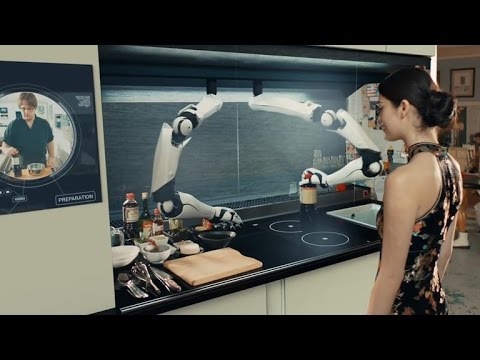In this intricately detailed photograph set against a gray background, we see a futuristic kitchen scene dominated by a young woman, likely Asian, positioned on the far right. Her black hair is neatly tied into a bun, and she is adorned in a tight, sleeveless vintage-style black dress accentuated with red, green, and golden foil details. The kitchen counter, possibly a stove, is sleek and black with white-trimmed burners and several cooking items like a cutting board, silverware, and bowls arranged on it. Above the counter, two robotic arms, white with black elements, are installed, with one holding a bottle, perhaps of wine or soy sauce. On the left wall, there is a screen displaying futuristic cybergenic visuals, reinforcing the sense that this scene is set in a technologically advanced future. Additionally, a framed picture of a man in a kitchen hangs on the left of the counter, contributing to the overall ambiance of the image, which appears to be a still from a film or commercial.